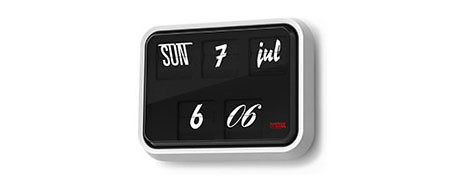This image features a computer-generated digital clock with a sleek, black oblong face encased in a thick, white plastic frame. The clock's display shows the day "S-U-N" for Sunday in white script text on the top left, a large number "7" in the middle indicating the date, and "J-U-L" for July written in lowercase script on the right. At the bottom of the display, the time is shown as "6:06" with a small, unreadable red mark next to it. The image is viewed slightly from the right, allowing a glimpse of the case’s side, which adds to the overall modern and digital aesthetic of the clock. The black face of the clock and the white text create a stark, easy-to-read contrast, further emphasizing its minimalist design.